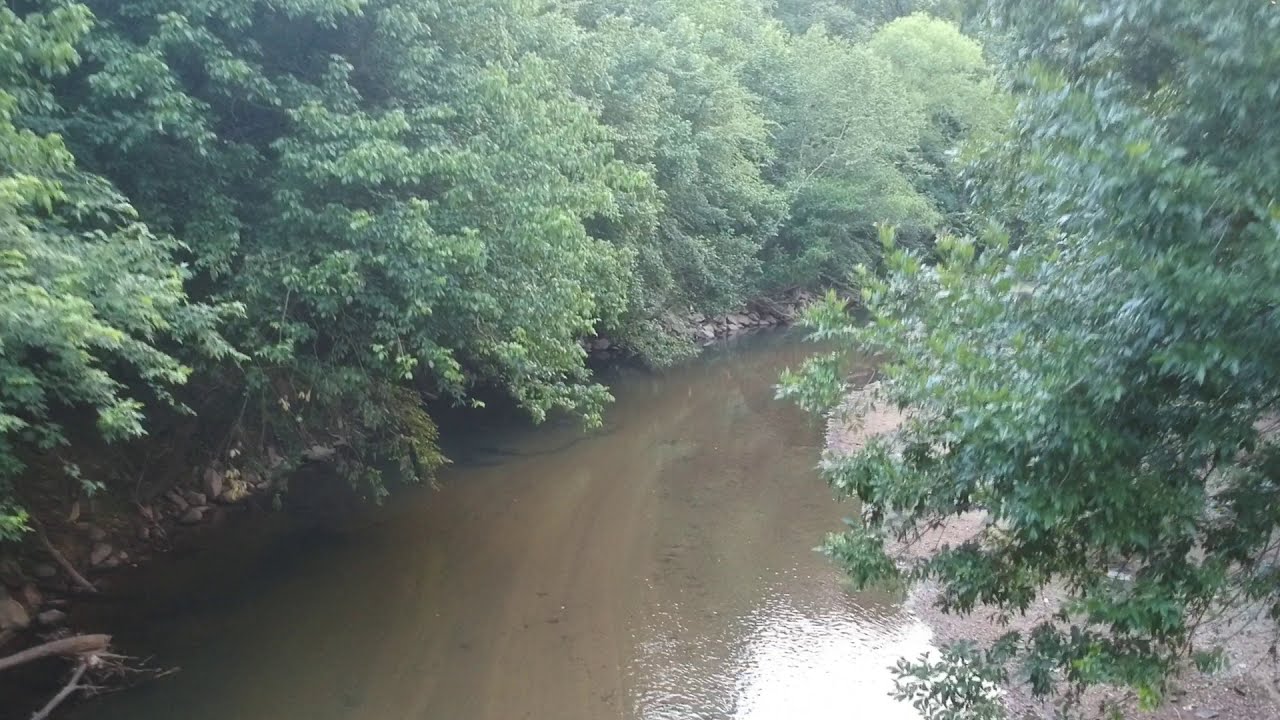This horizontally aligned rectangular picture, taken during the daytime, captures a serene, narrow creek with shallow, brown water flowing through the center. The dense area of trees on either side creates a canopy of green leaves, with numerous branches hanging over the water, casting intricate reflections. The creek’s banks, ascending on both sides, are lined with large rocks and exposed tree roots, partially covered in brown dirt. Toward the center at the bottom of the image, there’s a bright reflection from the sun on the water’s surface, indicating daytime illumination. Despite its somewhat blurry and slightly out-of-focus nature, the image showcases the creek’s clear waters, revealing the striations of sand and mud beneath. Although vibrant and full of greenery, the scene is devoid of visible wildlife, focusing solely on the natural elements of the trees and water. The upper right-hand corner is particularly dense with green leaves, adding to the lush surroundings, and the lower left-hand corner features some bare branches jutting out, enhancing the rustic and untouched feel of this tranquil setting.